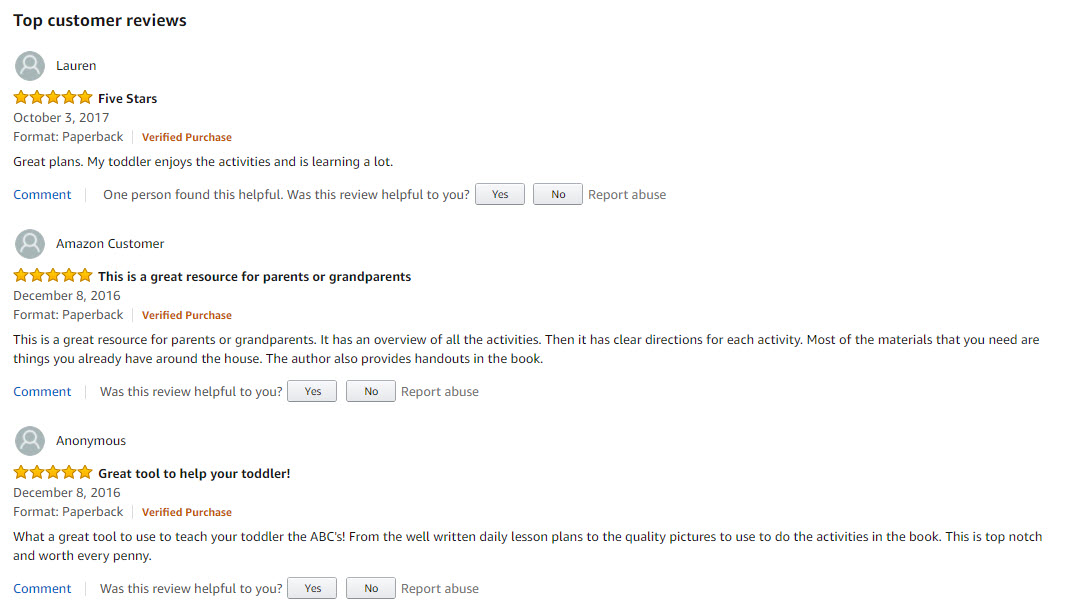This image showcases a webpage with Amazon customer reviews for a particular product. At the top, "Top Customer Reviews" is prominently displayed. Below this heading, there is a circle icon with a person inside it, labeled with the name "Lauren." Next to it, five stars are filled in with a yellowish color, signifying a five-star rating. The review title reads "Five Stars," and it is dated October 3, 2017. The format specified is paperback, verified purchase. Lauren's review states, "Great plans. My toddler enjoys the activities and is learning a lot." There is an option for readers to comment on the review, and it indicates that one person found it helpful. Readers can also select "Yes" or "No" for whether the review was helpful and have the option to "Report abuse."

Below Lauren's review, another review follows. It also features a circle icon with a person inside it, tagged "Amazon Customer." This review, rated with five yellow stars, has the title "This is a great resource for parents or grandparents," dated December 8, 2016. The format is again paperback, verified purchase. The text details that the book is a valuable resource for both parents and grandparents. It includes an overview of various activities along with clear instructions for each activity. Most materials needed are common household items, and the author also provides handouts within the book.

The third and final review on the page features an unidentified reviewer tagged as "Anonymous," with a five-star rating displayed below the icon. The headline reads "Great Tool to Help Your Toddler." The review text praises the book as a fantastic tool for teaching toddlers the ABCs, highlighting the well-written daily lesson plans and quality pictures. It concludes by affirming that the book is top-notch and worth every penny.